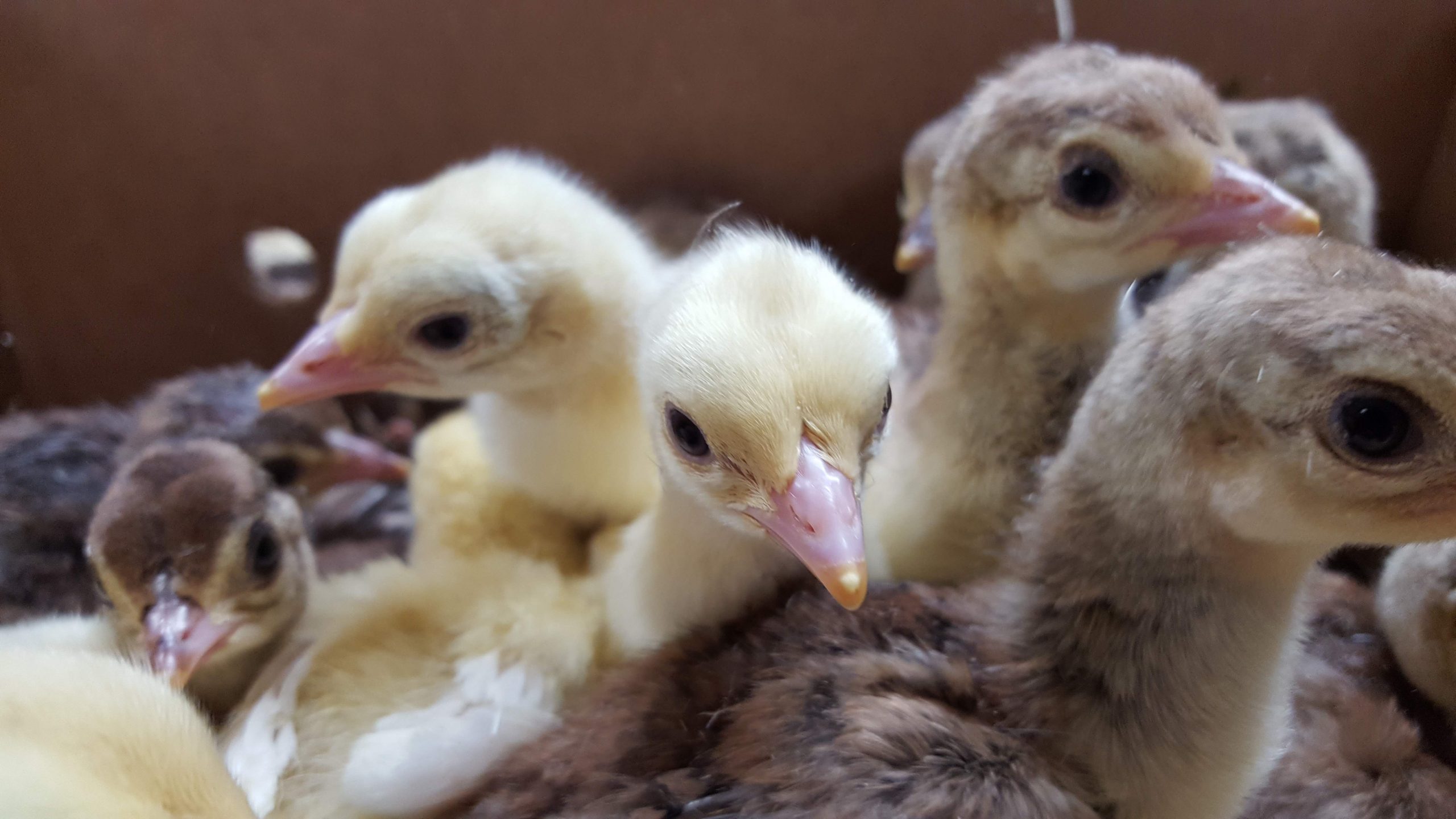This image is a close-up photograph of a group of baby birds, possibly a mix of chicks, turkeys, or ducklings, inside a box or hutch with a dark brown wooden background. The scene features a mix of yellow and brown baby birds, mostly with black eyes and pink beaks. At the center, two yellow chicks with pink beaks and orange tips are prominently visible. On the left side, there are slightly blurry brown chicks with similar pink beaks, while on the right, lighter brown chicks are noticeable, albeit one is partially obscured. Some birds have heads pointing in different directions, adding to a sense of dynamic disorder. There are also hints of white eggshell remnants on a few birds and blurry feather or shell casings in the foreground, suggesting a freshly hatched, lively environment. The image composition appears unusual, possibly indicating that it might be AI-generated, as the birds' bodies seem impossibly intertwined.